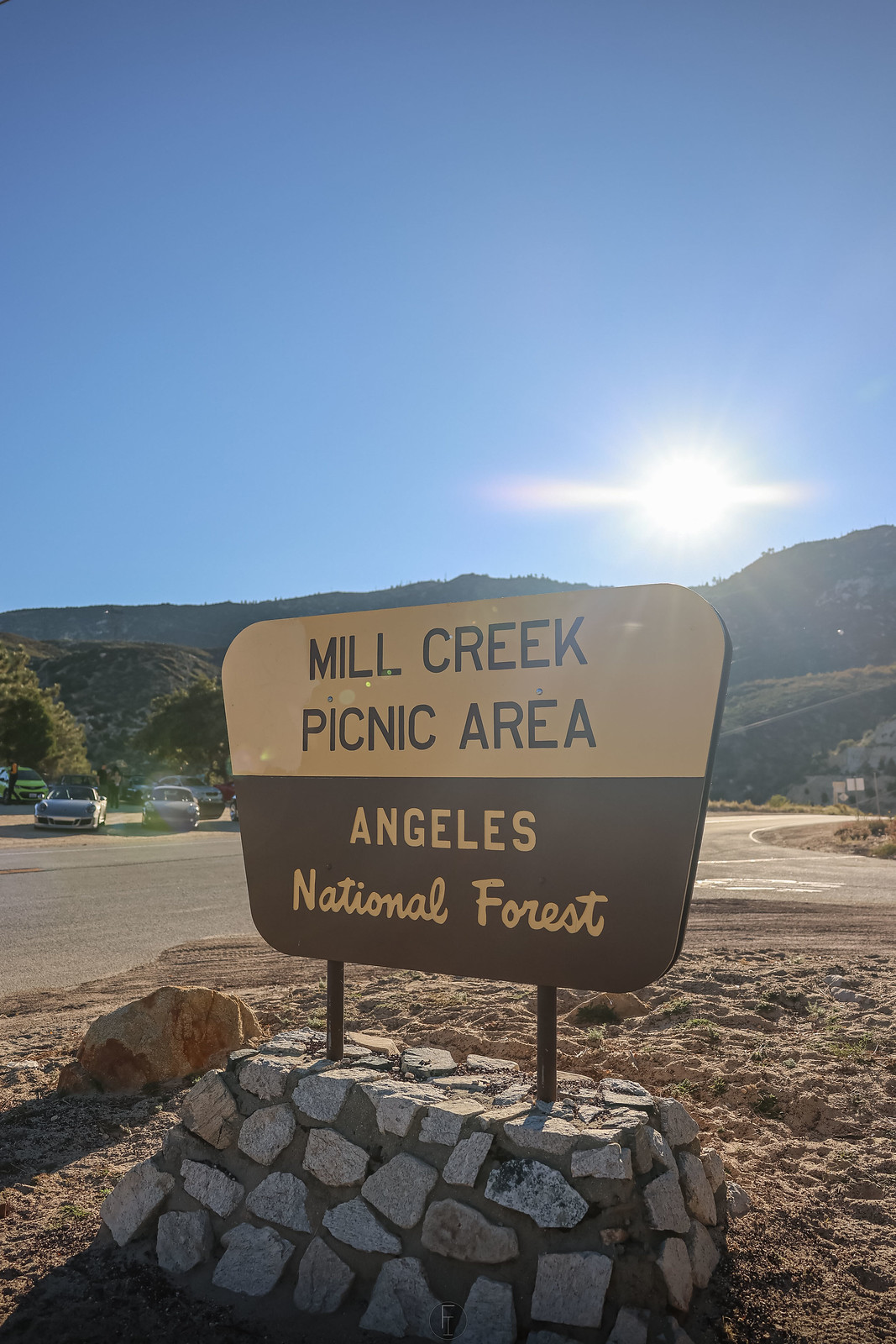This photograph captures a picturesque scene featuring a prominent roadside sign marking the Mill Creek Picnic Area. The focal point of the image is the trapezoidal-shaped sign with rounded corners, firmly mounted on a solid, stone and concrete base amidst a sandy gravel area. The sign is visually distinct, with its upper half in a tan or gold color bearing brown, capitalized letters that read "Mill Creek Picnic Area." Below, the sign transitions to a brown section with tan or gold letters stating "Angeles National Forest." 

The background reveals a serene, rolling hill covered in green vegetation under a bright blue sky during mid-morning. The sun is visibly rising, casting bright, streaky rays through a slight haze, adding a soft, ethereal glow to the scene. At the base of the hill, there are parked cars—some of which are high-end, like Porsches—hinting at a possible car show or meetup, with people potentially milling around. A road runs off to the left of the image, enhancing the sense of an accessible and welcoming outdoor area. The overall atmosphere is one of tranquil beauty, inviting visitors to explore and enjoy the natural surroundings of the Angeles National Forest.